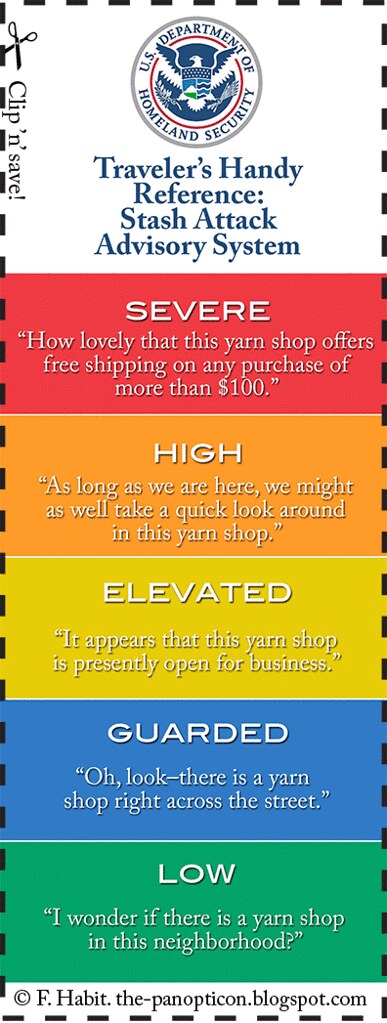The image is a digital screenshot styled to resemble a cover page, likely for a brochure, featuring an advisory system. At the top of the image, there's the U.S. Department of Homeland Security logo, featuring an eagle with a shield at the center. Above the logo, the text "Clip and Save" is written on a black border. Below the logo, in a white section, it reads "Traveler's Handy Reference Stash Attack Advisory System."

The advisory system is color-coded with various risk levels: 

1. "Severe" in a red box, followed by a caption: "How lovely that this yarn shop offers free shipping on any purchase of more than $100."
2. "High" in an orange box, with a caption: "As long as we are here, we might as well take a quick look around in this yarn shop."
3. "Elevated" in a yellow box, captioned: "It appears that this yarn shop is presently open for business."
4. "Guarded" in a blue box with the caption: "Oh look, there is a yarn shop right across the street."
5. "Low" in a green box, accompanied by the caption: "I wonder if there is a yarn shop in this neighborhood."

At the bottom of the image, a footnote contains a copyright symbol with the text "f.habit.thepanopticon.blogspot.com". The colors used prominently throughout the image include red, orange, yellow, blue, green, black, and white.